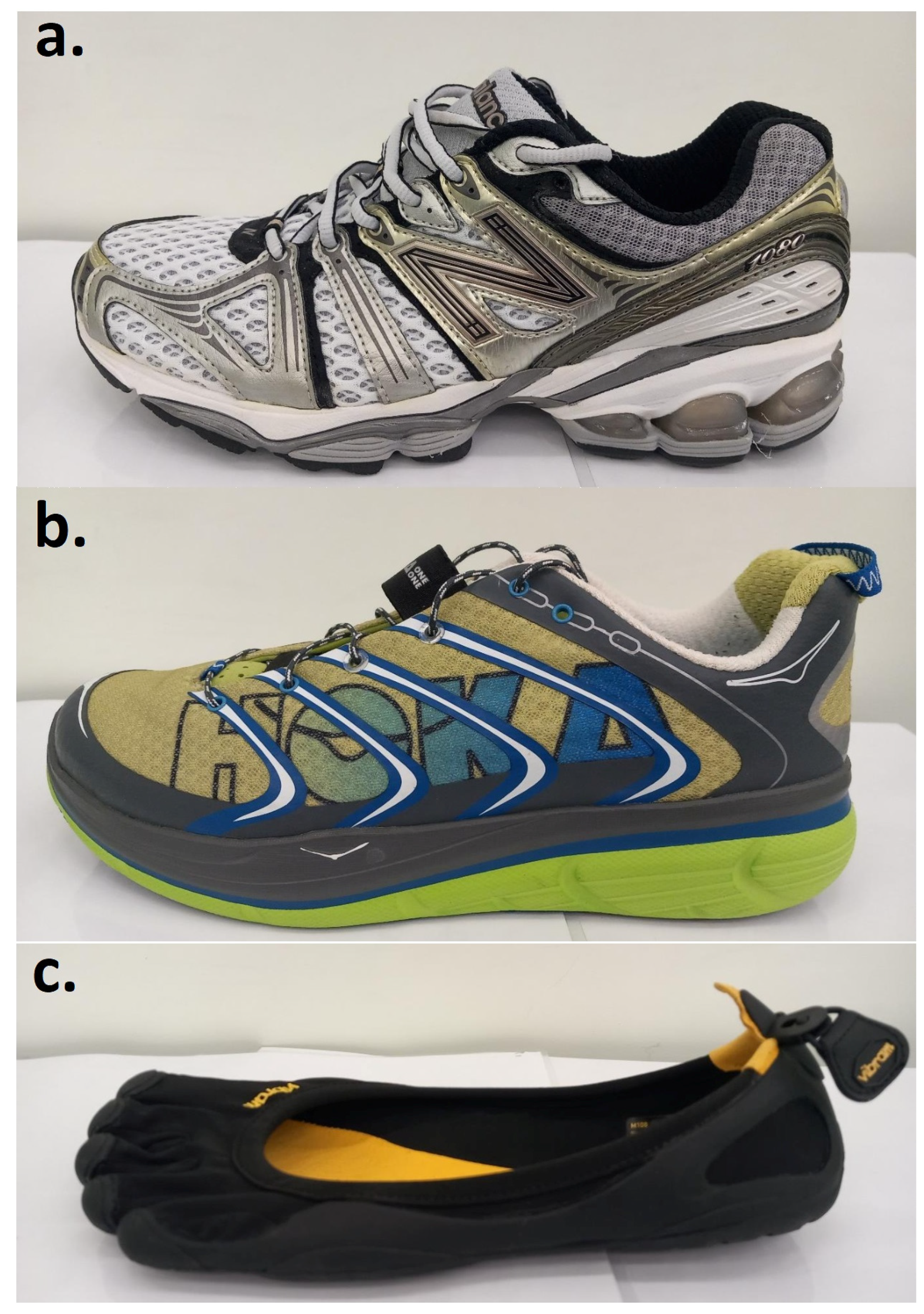This indoor, full-color image showcases three close-up photographs of different types of footwear, labeled A, B, and C in black lowercase text at the top left of each section. The photos are vertically aligned and appear to be arranged on a white shelf under artificial lighting.

In the top section (A), there's a men's New Balance running shoe presented from the left side. This shoe is predominantly gray with a hint of gold trim around the iconic large 'N' logo. It features white shoelaces, a black interior, a thick sole, and a mesh upper, reflecting a design suitable for running.

The middle section (B) displays a Hoka running shoe, identified by the block-style text "HOKA" in gold and blue letters on the side. This shoe is visually striking with its white diagonal stripes, blue accents, bright green sole, and multicolored design incorporating black, blue, and brown elements. The shoe is seen from the left side, highlighting its thick sole and athletic style.

In the bottom section (C) lies a unique black water shoe, shaped distinctly with defined toe sections, resembling a foot. It includes yellow insoles and a small heel tag for easy pulling. This minimalist shoe looks relatively less supportive and more designed for water-based activities or minimalist running. 

Each of these photos collectively provides a detailed comparison of varied footwear styles, suitable for different purposes ranging from traditional running to specialized water activities.